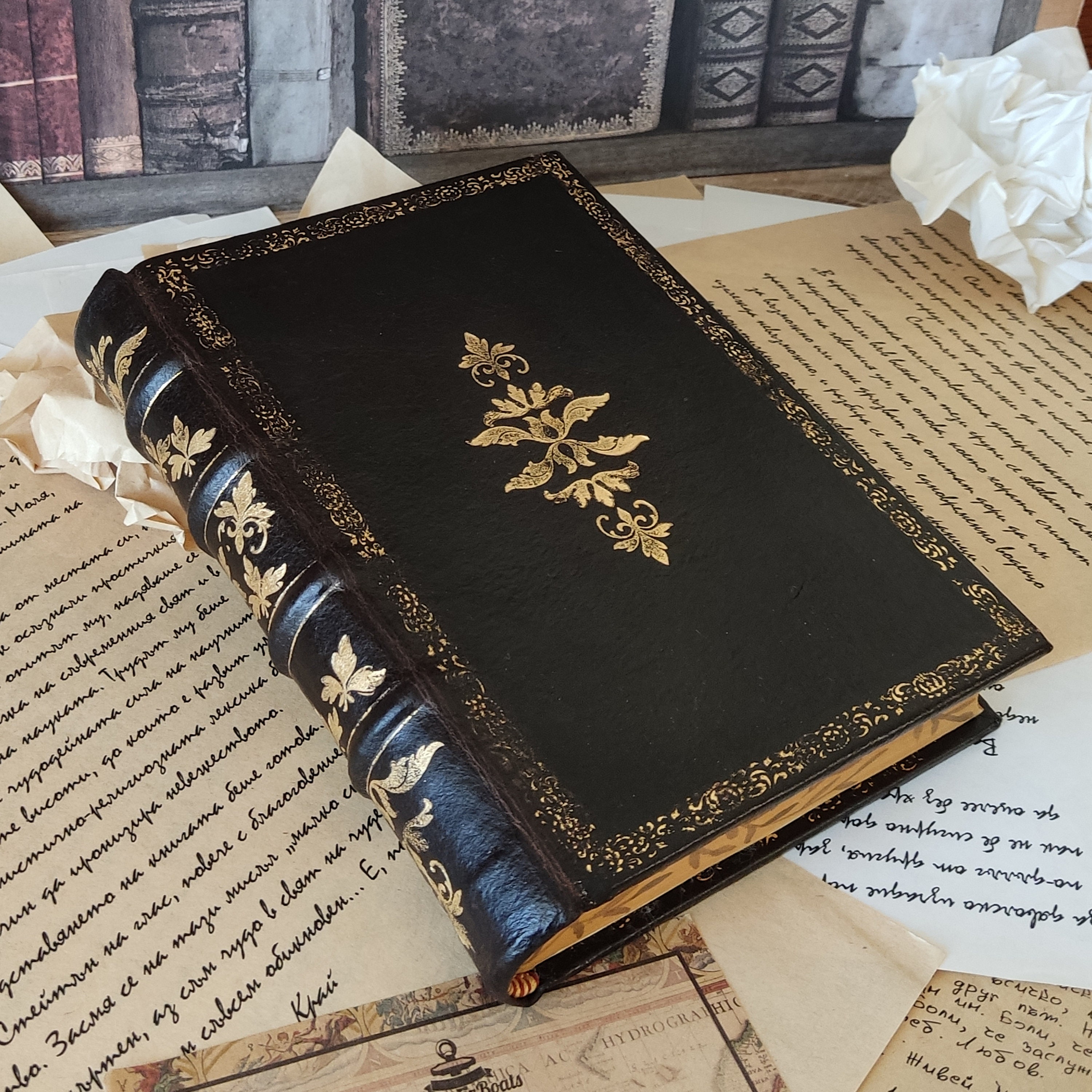This photograph captures a close-up of an old, black leather-bound book with a gold floral and leaf motif in the center of its ornately decorated front cover. The book, which appears to be in fairly good condition despite its age, is adorned with gold leafing that beautifully accents its spine and the edges of the front cover. It rests on a table cluttered with numerous letters and notes, some on brown parchment paper and others on white stationery. The letters, written in cursive script and possibly in a different language, add to the historical ambiance of the scene. A distinguishable piece among the letters features stationery with a logo that mentions "boats" and "hydrographic." In the upper right corner of the image, there's a crumpled piece of paper. The background reveals a shelf filled with old books, further enhancing the vintage atmosphere of the photograph.